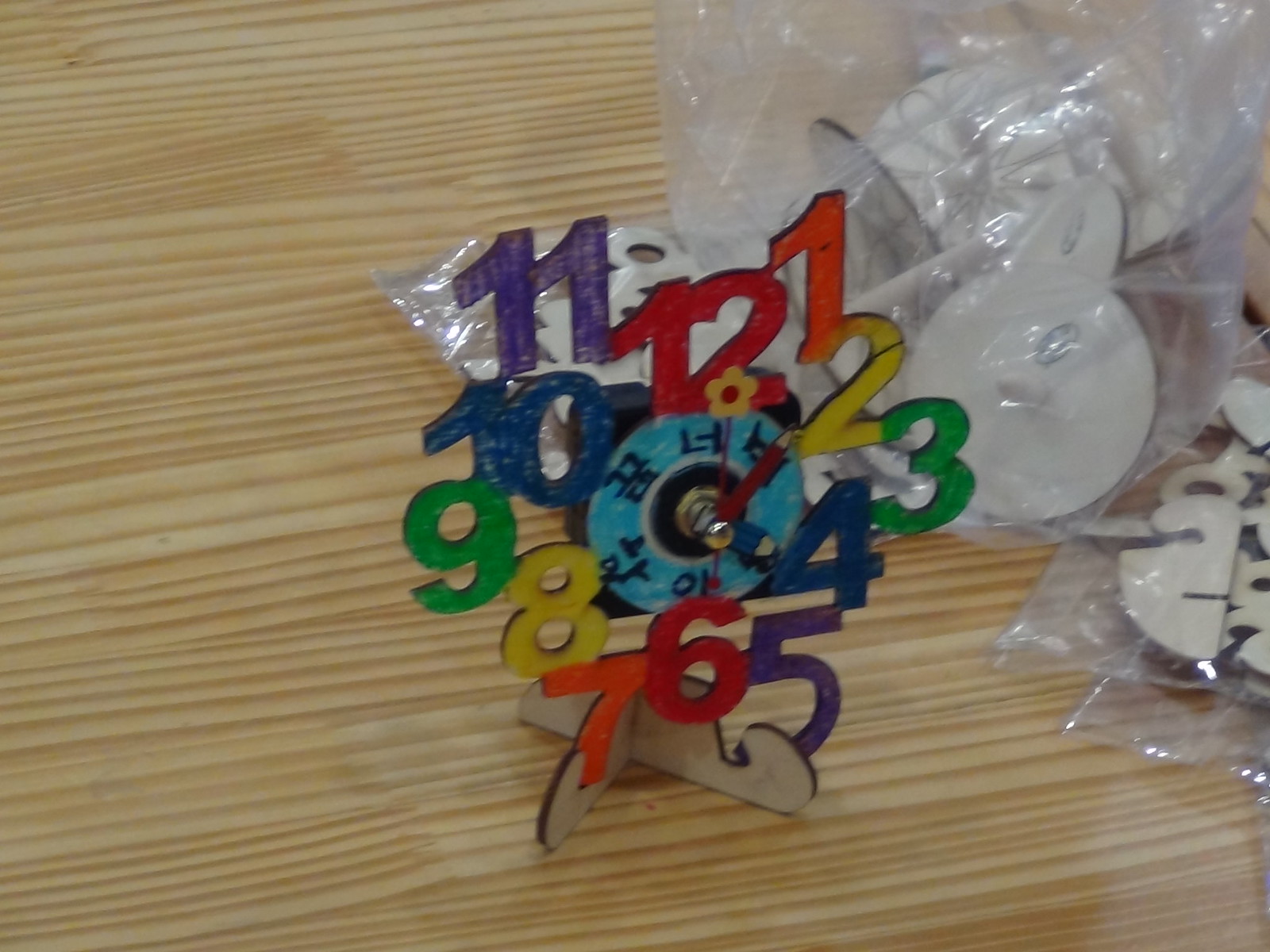This photo showcases an artistically designed, eclectic clock. The clock's face is unconventional, with numbers 1 through 12 floating around the center in varying heights and lengths without being enclosed by a traditional frame, creating an impression of movement and whimsy. The numbers are painted in a repeating color pattern: orange (1 and 7), yellow (2 and 8), green (3 and 9), blue (4 and 10), purple (5 and 11), and red (6 and 12). At the center of the clock is a small circular base with a light blue background featuring black Chinese or Japanese lettering, from which gold-like knob holds the clock's hands. The clock hands include a red pencil-shaped hour hand, a shorter and wider blue pencil-shaped minute hand, and a small red seconds hand adorned with a yellow flower at the tip. The clock rests on a light brown wooden table with noticeable dark brown grains, adding to the rustic aesthetic. In the top right corner of the photo, two plastic bags containing white items can be seen.